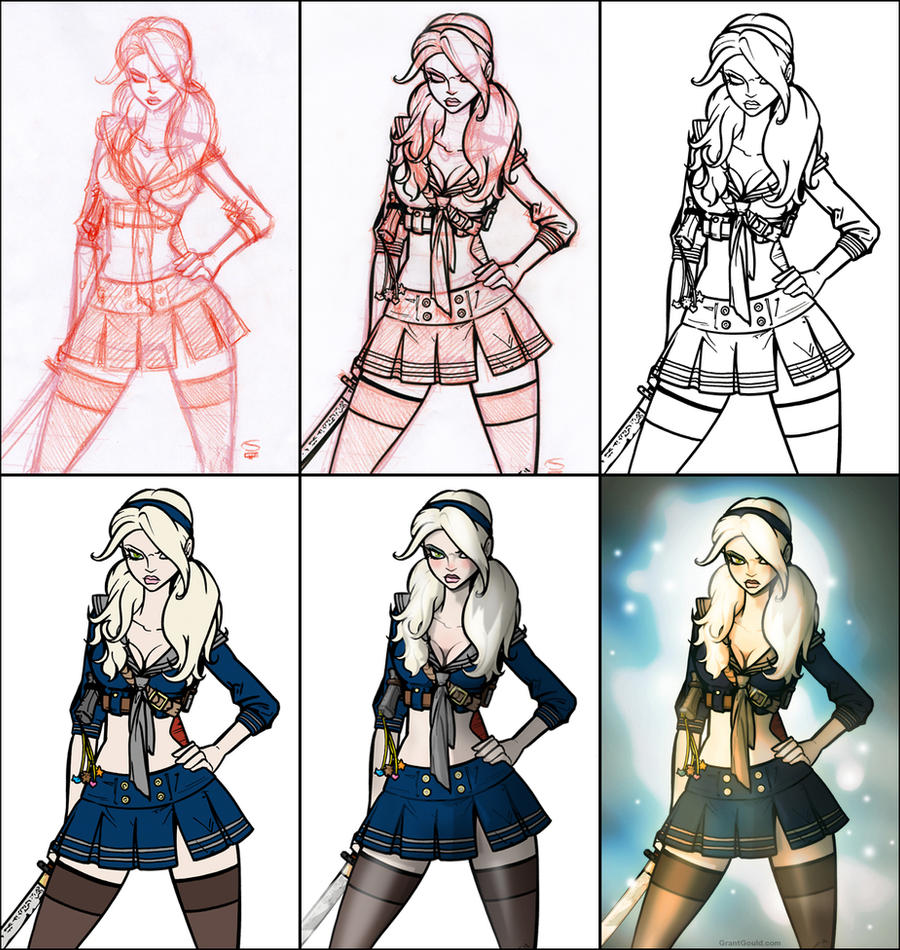The image depicts the progressive stages of creating an anime-style drawing of a young woman, arranged in two rows of three pictures each, documenting the transformation from initial sketch to final illustration. In the top left, the first stage is a red outline on a white background, showing the basic form of the woman, who has long hair, a pleated miniskirt, a halter top, and thigh-high hose, holding a sword by her side. Moving to the center image of the top row, the sketch becomes more defined with additional dark red outlines overlaying the initial red. By the top right, the drawing features a clean black outline without any red sketch marks. Transitioning to the bottom row, the fourth image introduces flat color fills for her blonde hair, blue outfit, skin, and sword. In the fifth image, shadow details are added to enhance depth and realism. The final illustration on the bottom right presents the woman fully rendered with vibrant colors, detailed shadows, and highlights. She stands with her legs slightly apart in an assertive pose, her hand on her hip, and gazes upward. She sports a blue dress, leggings, and a headband, with her midriff exposed and a little bow at the middle of her shirt. The background behind her glows with touches of light dots and a gradient from dark to light, adding a dramatic effect to the completed artwork.